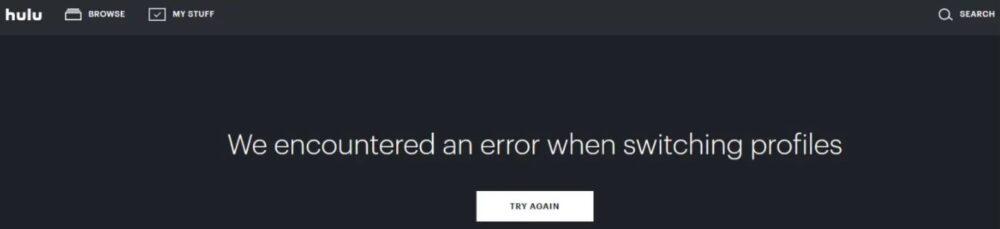The image is a narrow, horizontally-oriented rectangle with a black background. In the upper left corner, the Hulu logo is displayed in white. Adjacent to it on the right are the options for "Browse" and "Buy Stuff." On the far right, there is a search icon accompanied by the word "Search," indicating an option to click and search within the platform. The central portion of the image has a prominent error message. It reads "We Encountered an Error when Switching Profiles," in white text, indicating a technical issue. Directly beneath the error message, a horizontally-oriented, white rectangular button is centrally positioned. Within this button, "TRY AGAIN" is inscribed in black, uppercase text, urging the user to attempt to fix the issue by clicking.

This detailed, cleaned-up caption provides a clear and thorough description of the image, encompassing all the essential elements.